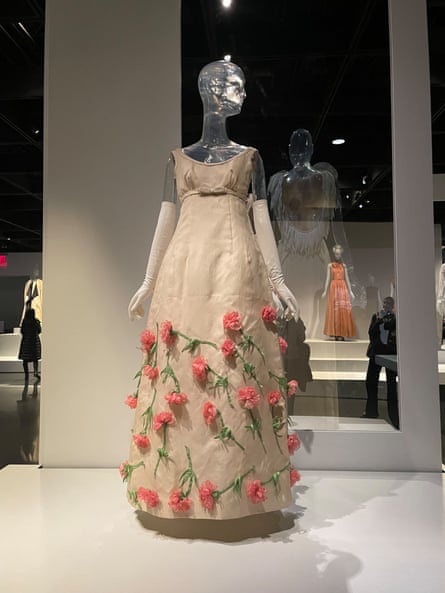The image captures an exquisite display in a formal wear shop. The central focus is a unique transparent mannequin, resembling crystal, elegantly dressed in a light tan floor-length gown adorned with intricately sewn pink flowers and green leaves and stems near the bottom. The mannequin's ensemble is completed with light cream-colored gloves extending from its fingertips to just above the elbow. In the background, beyond a glass window leading to another room, there's a figure—possibly a real person or a mannequin in a tuxedo. Further back, a female mannequin stands on a two-step white stage, elegantly dressed in a sleeveless light orange dress. The setting features all-white walls and steps, contributing to the pristine atmosphere. To the left, a real person is visible, walking away from the camera, and another mannequin, attired in a gray and yellow outfit, stands on stage. The image also captures various soft hues, including white, pink, tan, green, black, and light orange, enhancing the overall aesthetic. Shadows from the mannequins lend depth to the scene, and an exit sign is partially visible near the left edge of the photo.